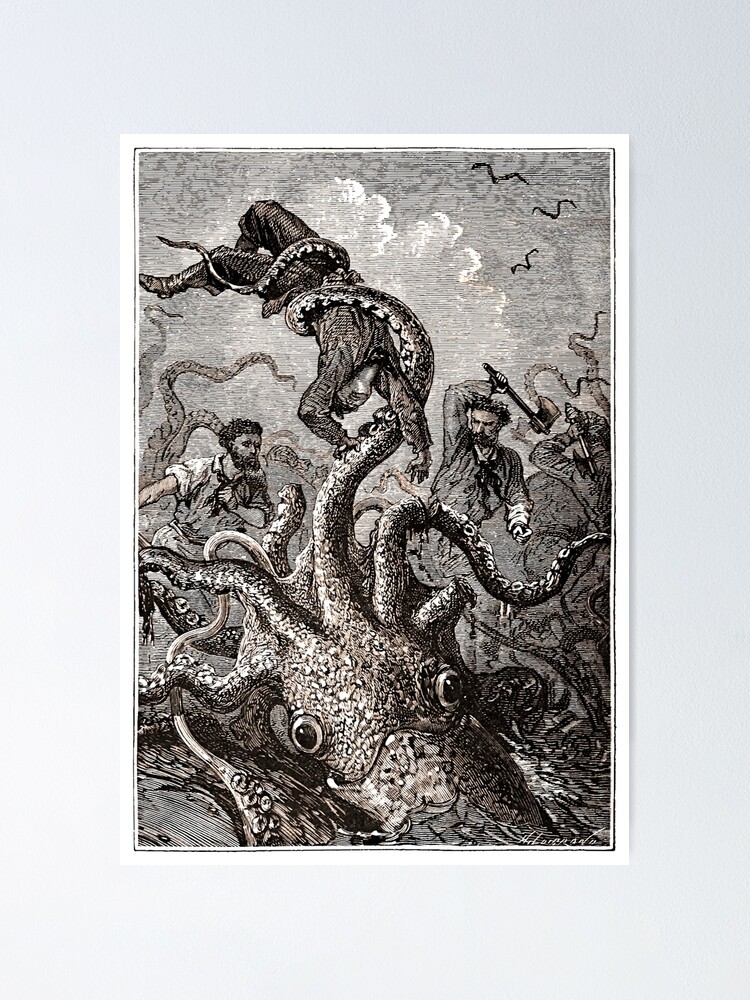The image is an intricately detailed, black and white pen and ink etching, enclosed in a very light gray matted frame with a beveled edge. The focal point is a monstrous, octopus-like sea creature with sinister, large black eyes positioned at the lower part of its head. The creature's numerous tentacles writhe menacingly through the scene. One tentacle hoists a man upside down by the waist, while another stretches towards the right, where a man wielding an axe prepares to strike. To the left, a terrified man appears to be in full flight, trying desperately to escape the chaos. The background is a stormy expanse of gray clouds, punctuated by bats—possibly mistaken for birds—swooping through the top right. This artistic rendering vividly captures the dramatic and perilous confrontation between the men and the sea monster.